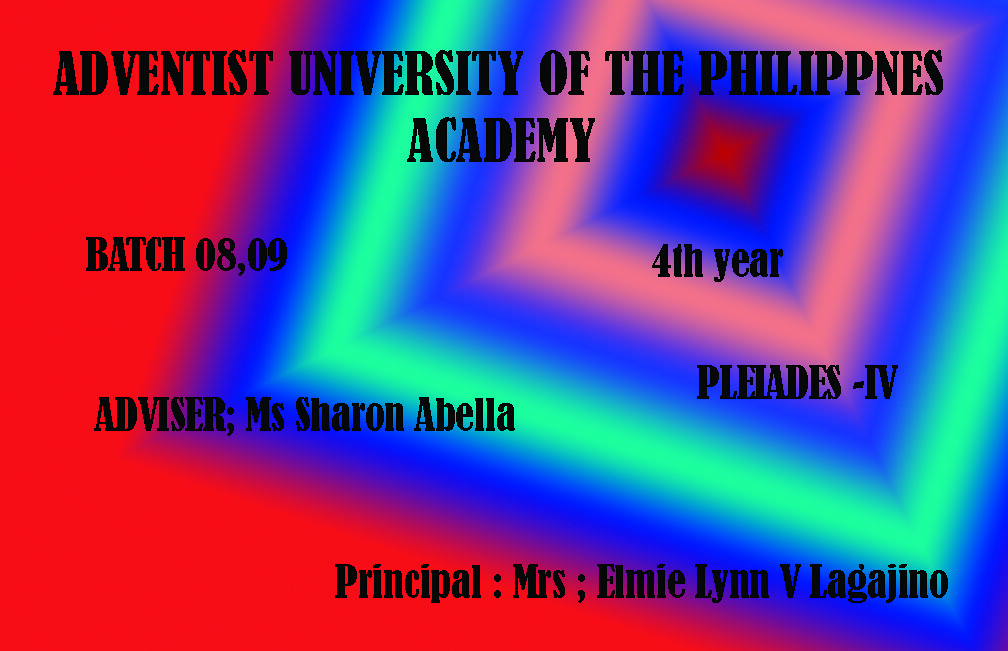The image displays a colorful, multi-layered geometric design featuring concentric squares. Starting from the center, there is a red square, followed by progressively larger squares in blue, pink, blue, mint green, and again blue. The outermost borders are mostly a vibrant red. In the top part of the image, bold black text reads "Adventist University of the Philippines Academy," though there is a missing "I" between the "P" and "N" in "Philippines." Below this title, the text is divided into two sections: on the left, it reads "Batch '08, '09," and on the right, it says "Fourth Year." Below these lines, it reads "Advisor: Ms. Sharon Abella" on the left and "Pleiades IV" to the right. At the bottom of the image, the text states "Principal: Mrs. Elmi Lin V. Lagugino."